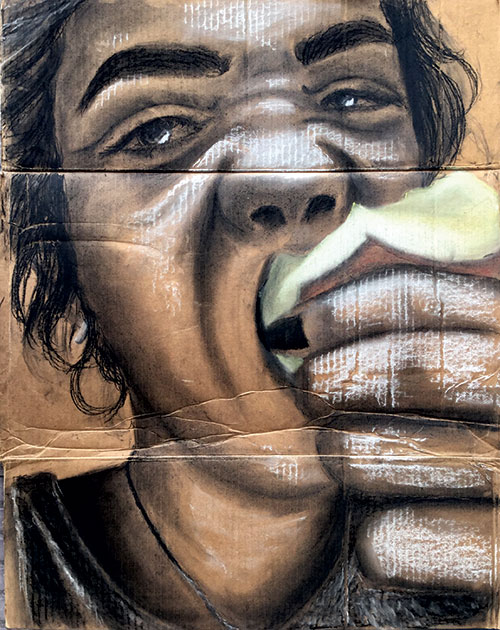This artwork is a vibrant multi-color artistic piece painted on cardboard. The vertically rectangular image captures a striking close-up of a person who appears to be a woman with dark, shaggy, curly hair and thick black eyebrows. The painting details her mid-bite into a partially-eaten apple, which she holds in her right hand. Her mouth is open around the apple with her nose and cheeks bunched up, showing a range of expressions.

The artwork features notable white highlights on her nose, cheeks, forehead, and fingers, contrasting sharply with her brown-tan skin tone, likely for artistic effect. She is depicted wearing a black tank top and a black necklace, adding to the depth and detail of the scene. 

The cardboard canvas has visible creases, folds, and horizontal seams, suggesting it was folded up and used in a raw, torn state. The background is a burnt orange hue, peeking through sparsely and adding warmth to the composition. The image's handling of folds, texture, and color creates a depth and dynamism, emphasizing the intense and immediate nature of the moment captured in the artwork.